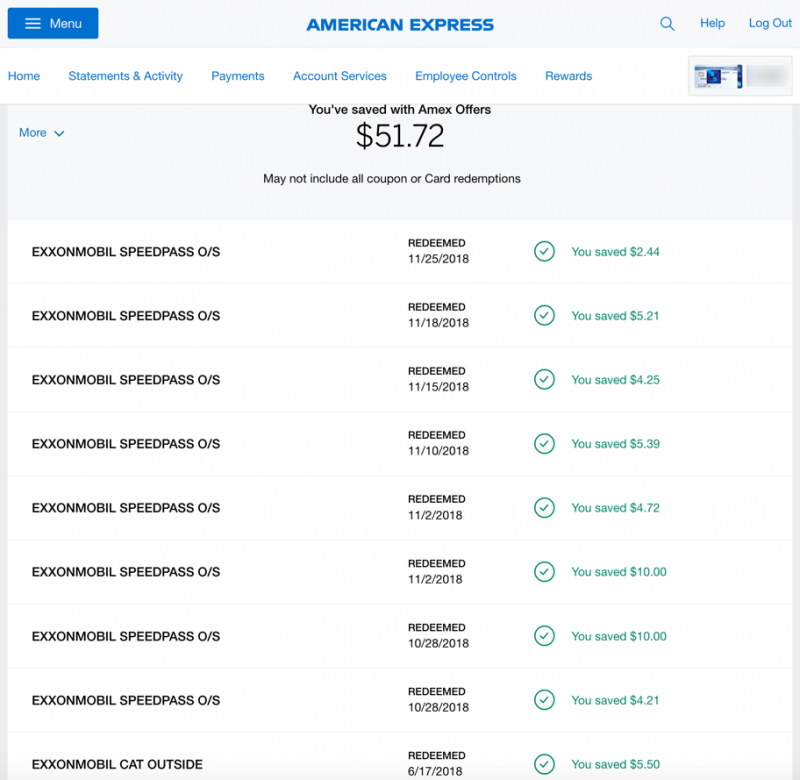This image features a detailed view of an American Express account webpage. Dominating the top of the page are the large, bold blue letters spelling "American Express." On the left side, a blue box houses the main menu, containing several navigational links such as "Home," "Statements and Activity," "Payments," "Account Services," "Employee Controls," and "Rewards." 

Situated on the right side of the header are icons and options for search, help, and logging out. Below the header, there is a section in gray with a drop-down menu marked "More."

Prominently displayed on the right side of the page is an image of an American Express card. Directly beneath this, a message indicates that "$5,172" has been saved with Amex offers, though it may not include all coupons or card redemptions. 

Further down, the page details the user’s activities for the month, with notable transactions including multiple entries from Exxon Mobil SpeedPass OS. The dated entries from 2018 include activities on 11/25, 11/18, 11/15, 11/10, 11/2, and 10/28, listing corresponding savings in green text, which include amounts like $244, $521, $425, $539, $472, $10, and $550.

The lower segment of the webpage is cut off, hence, the subtotal for the savings and activities is not visible.